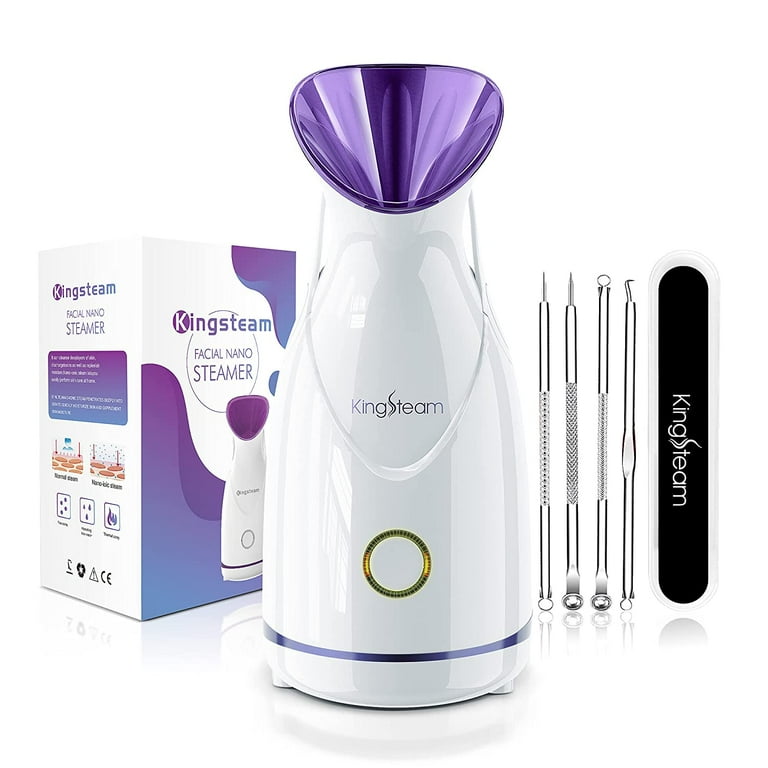The image is a staged, full-color, promotional photograph taken indoors with artificial lighting. The background is predominantly white, serving as a seamless backdrop. At the bottom of the image, there's a faint reflection of the items.

On the far left, there is a white and purple cardboard box displaying the Kingsteam Facial Nano Steamer, complete with a picture of the steamer and some instructional text. In the center of the image is the Kingsteam Nano Steamer itself. The steamer features a white plastic body with a distinctive purple mouth opening at the top, angled outwards. A golden circular button sits below the opening, surrounded by a brass ring, adding to its sleek design.

To the right of the steamer are four metallic, dentist-like tools, likely intended for skincare purposes such as extracting blemishes. These tools vary in shape and include needle points, metal cushions, and ball shapes, each with their own gripping sections designed for different functions.

On the far right, there is a vertical black tube with the word "Kingsteam" written along its length in white letters. This tube likely serves as a holding case for the skincare tools. The detailed arrangement and professional lighting highlight the product's features, emphasizing its utility and aesthetic appeal, making the image suitable for advertising or product listings.